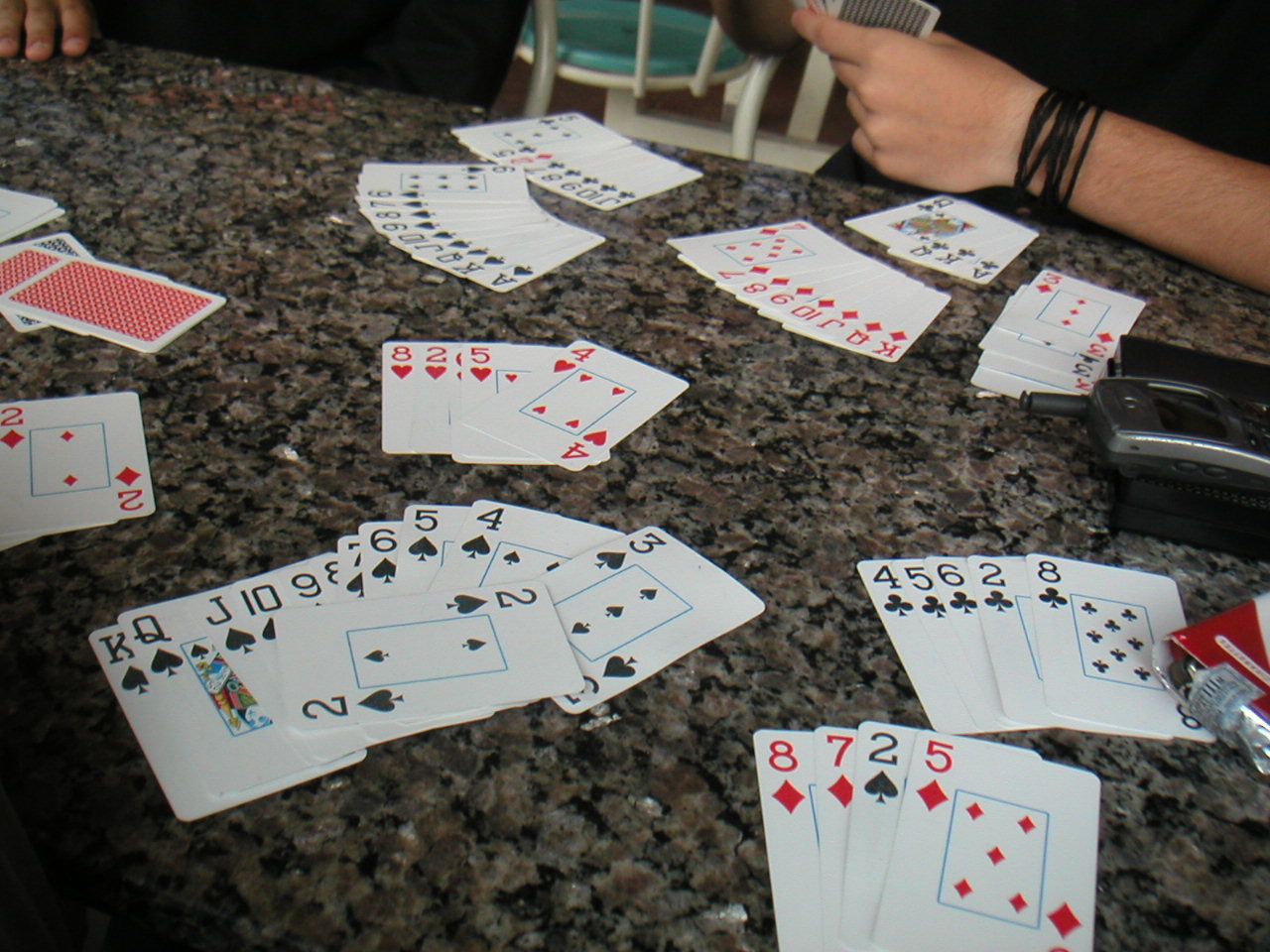This image captures a moment on a stylish granite countertop, featuring an intricate pattern in shades of brown, silver, charcoal, and black. A person, visible only by their arm and hand, extends from the top right corner of the frame. Their arm, adorned with multiple black bracelets, hovers over the countertop as they hold a hand of playing cards. 

The surface is scattered with various cards—noticeably, an 8 of hearts, a 2 of hearts, a 5 of hearts, and a 4 of hearts grouped together. Specific suits cluster nearby, with bunches of spades and clubs adding to the mix. 

In the background, a teal chair with a distinct white back adds a pop of color to the setting. On the right-hand side of the countertop, a partially visible red pack of cigarettes, slightly open to reveal a lighter inside, catches the eye. Next to it, an older model house phone rests on a black charger, completing the scene.